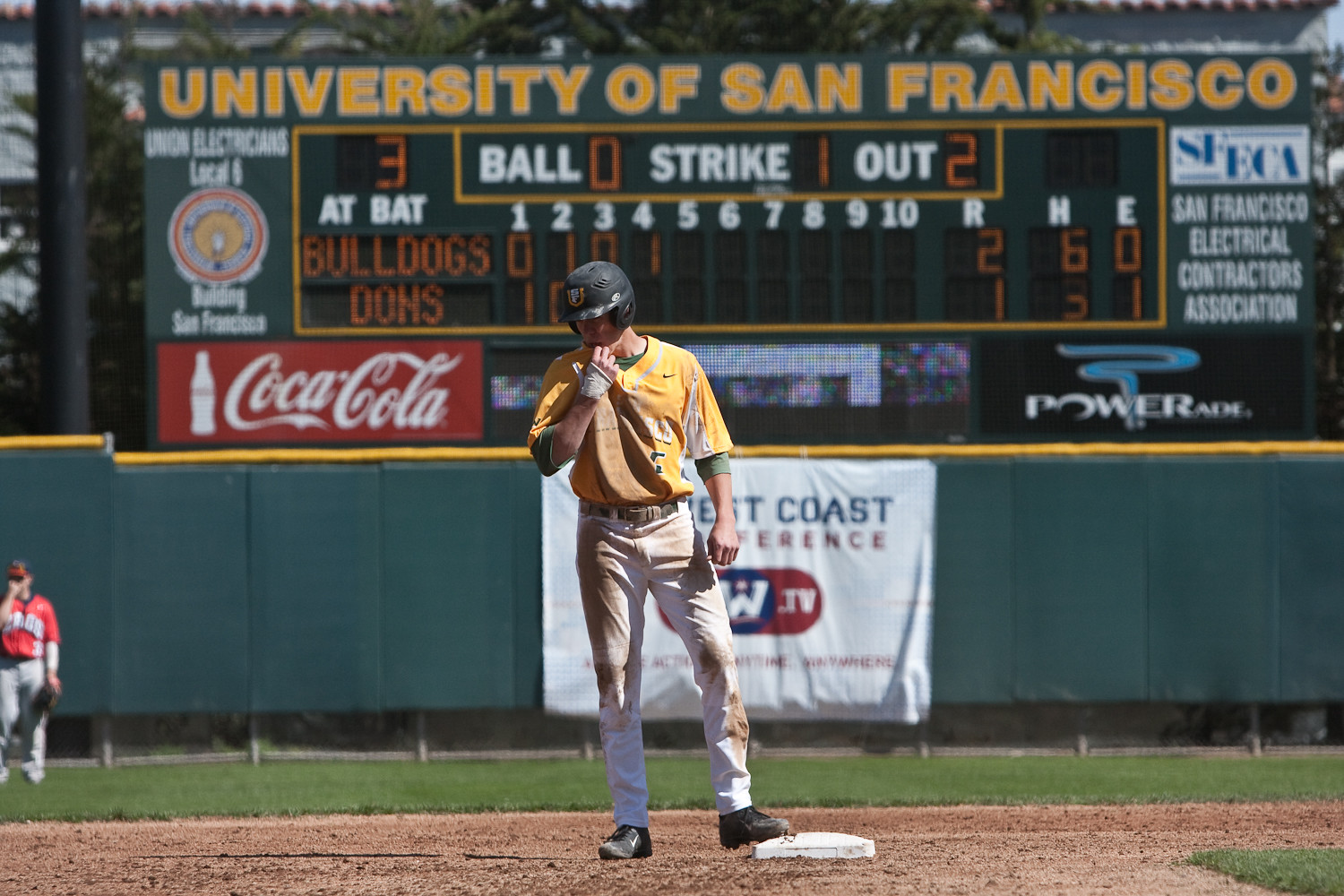This detailed image captures a moment during a baseball game, with a primary focus on a player positioned on a base. The player, wearing a yellow jersey with a black Nike logo on the top left and a green undershirt, stands firmly with his left foot touching the white base. He is sporting a black helmet and white pants, heavily soiled with dirt, held up by a belt. The player is also equipped with black cleats featuring a visible white Nike logo, and a bandage wrapped around one of his hands. In the background, a large scoreboard reads "University of San Francisco," displaying the current game details: at bat three, Bulldogs ball zero, strike one, out two, run to home six, and an error count of zero. Sponsors’ advertisements such as Coca-Cola, Powerade, and the San Francisco Electrical Contractors Association adorn the scoreboard. Another player can be seen in the outfield, dressed in a red jersey, gray pants, and a black and red hat. The scene is set with a rich ambiance of the baseball field, complete with dirt, tension, and the excitement of the game.